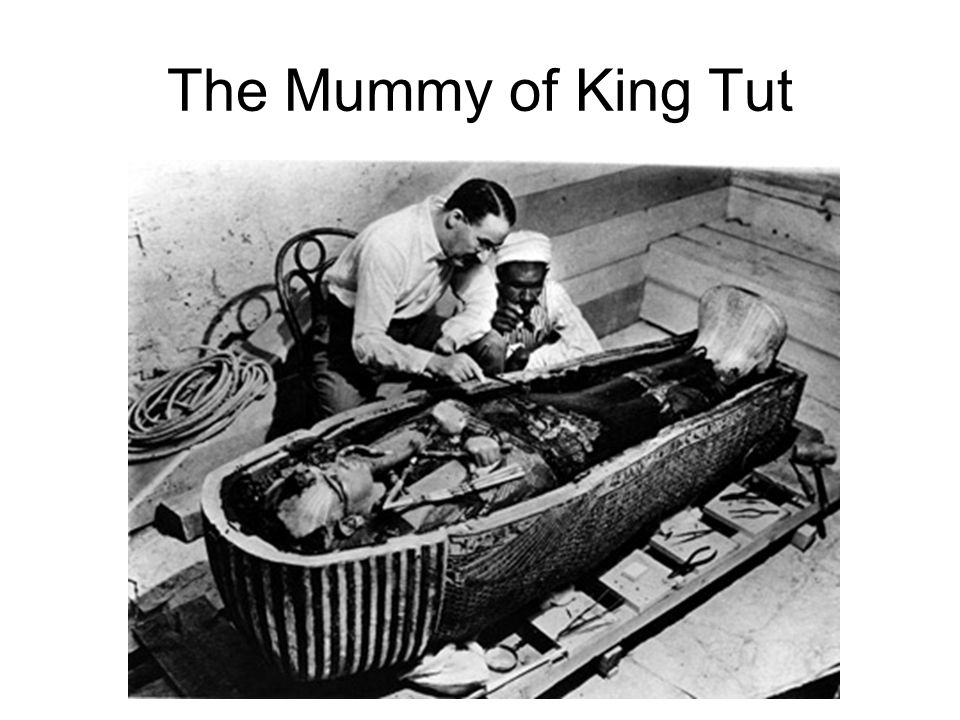In this black and white photograph, with the text "The Mummy of King Tut" displayed prominently at the top in black lettering, we witness an intriguing scene set against a white background. The focal point of the image is the open sarcophagus at the bottom center, containing the mummy of King Tut, with the head positioned to the left and the feet to the right. The sarcophagus rests upon wooden structures, possibly part of an archaeological setup. Surrounding it are various tools, indicative of an excavation site.

Two men are closely examining the mummy; one, seated on a wooden chair and clad in a button-up shirt, has dark hair neatly parted to the side. The other man, wearing a white cap and matching white shirt, is squatting beside him, possibly in observant conversation. Notably, there is a coil of rope behind them, contributing to the overall authenticity and historical context of the scene. Above and to the right of the sarcophagus, a staircase is visible, adding depth to the setting. The image, reminiscent of an older photograph, is laid out in a manner that avoids overcrowding, with each object and figure well-positioned, evoking the style of a meticulously crafted PowerPoint presentation.